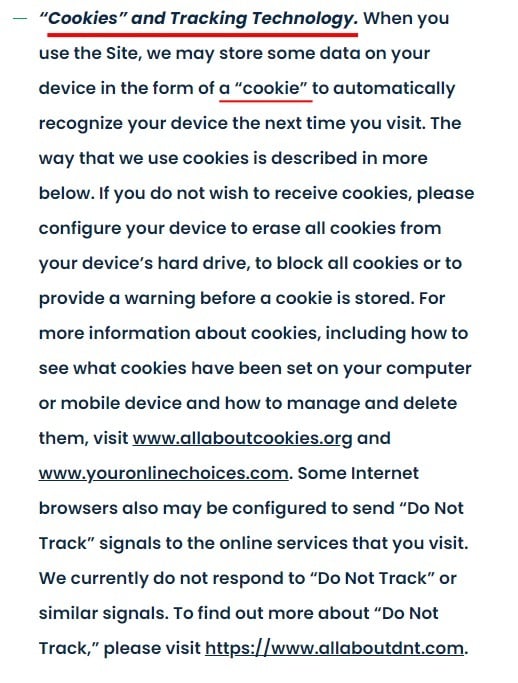The image features black text on a white background, without any borders. At the top, bold black text reads "Cookies and Tracking Technology," which is underlined in red. The text explains that by using the site, data may be stored on the user’s device in the form of cookies. The word "cookie" is underlined in red to signify its importance. The purpose of these cookies is to automatically recognize the user’s device during subsequent visits. The text further outlines that specific information on cookie usage is provided below.

It advises users who do not wish to receive cookies to configure their devices to erase all cookies from their hard drive, block all cookies, or provide a warning before a cookie is stored. For detailed information about cookies, including how to view, manage, and delete them, users are directed to visit www.allaboutcookies.org and www.youronlinechoices.com.

The text also notes that some internet browsers can be set to send "Do Not Track" signals to online services. However, the site currently does not respond to these signals. For more information on "Do Not Track," users are encouraged to visit https://www.allaboutdnt.com.